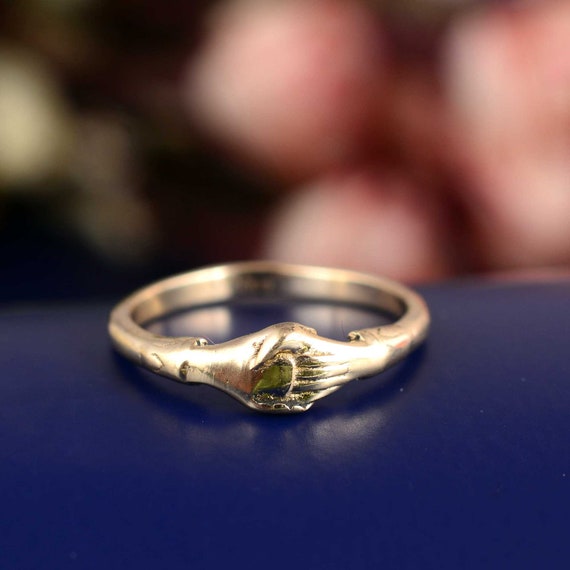The image showcases a small, handmade ring crafted from a silver metal, possibly brass or bronze, which appears cast. The ring features two clasped hands, possibly representing a handshake, with detailed cuffs where the wrists meet. The decorative clasped hands section looks slightly deformed, suggesting it may not have been perfectly positioned during casting. The band of the ring itself is plain. The ring rests on a deep royal blue surface, sharply in focus, while the background is blurred and filled with pink, red, and some greenish-black hues, possibly indicating flowers or fingers pinching something. The background fades into darker shades towards the left side. There appears to be some inscription on the inside of the ring, though it is out of focus and unreadable.